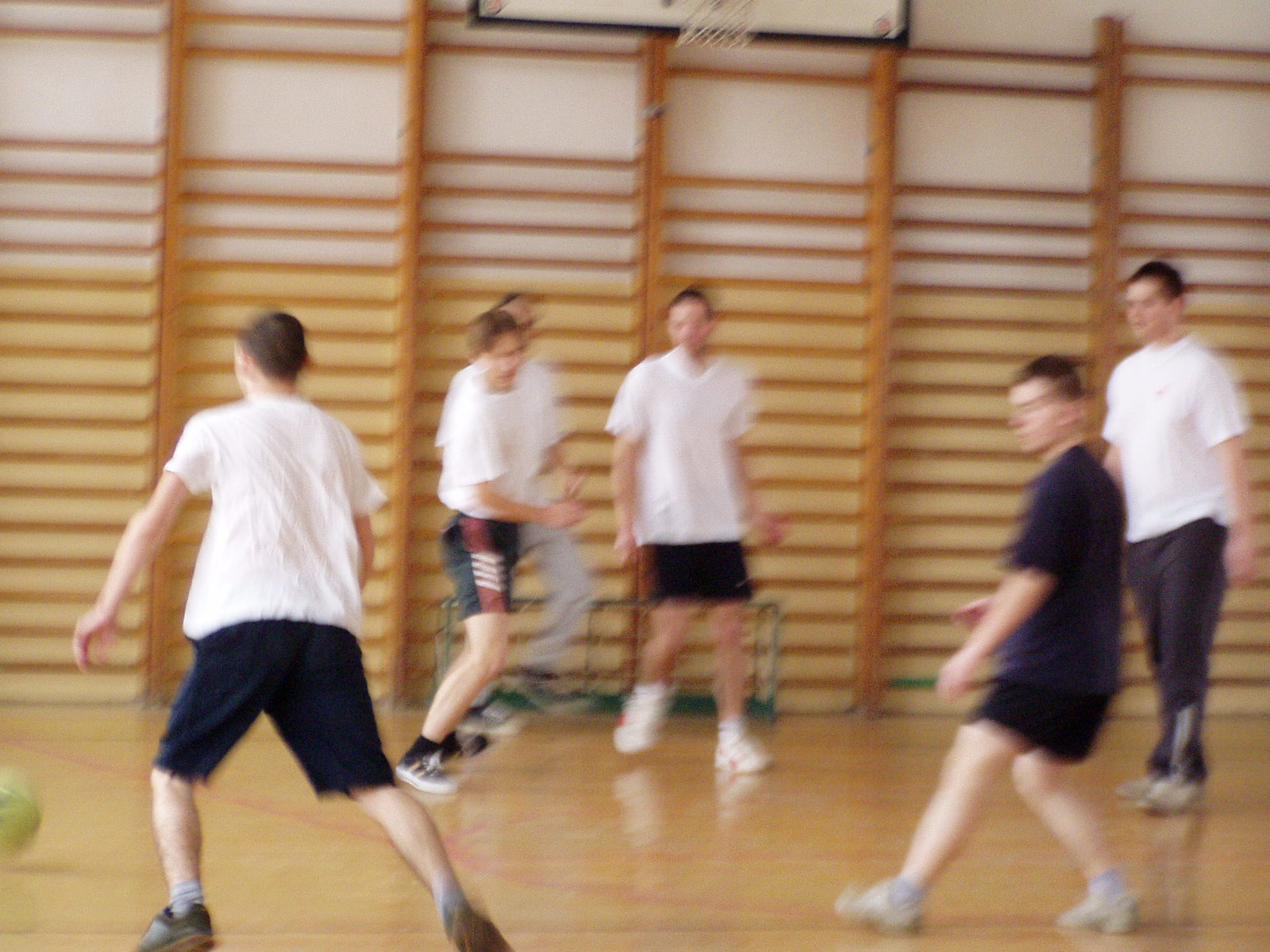The photograph captures a vibrant indoor gymnasium scene featuring six teenagers engaged in a game of basketball. Five of the boys are dressed uniformly in white t-shirts and black shorts, while a sixth boy on the right stands out in a black t-shirt and black shorts. One player is distinguished by wearing black long pants. The action is slightly blurred, suggesting dynamic motion as they play, with all eyes seemingly focused on a yellow basketball situated in the bottom left corner of the image. The gym floor, a highly polished and light-colored wood, gleams under the overhead lights. The back wall, painted yellow, features various wooden climbing frames and steel beams, adding a structured backdrop to the energetic scene unfolding on the court. The image captures a moment of anticipation and movement, reflecting the intensity and focus of the youths' game.